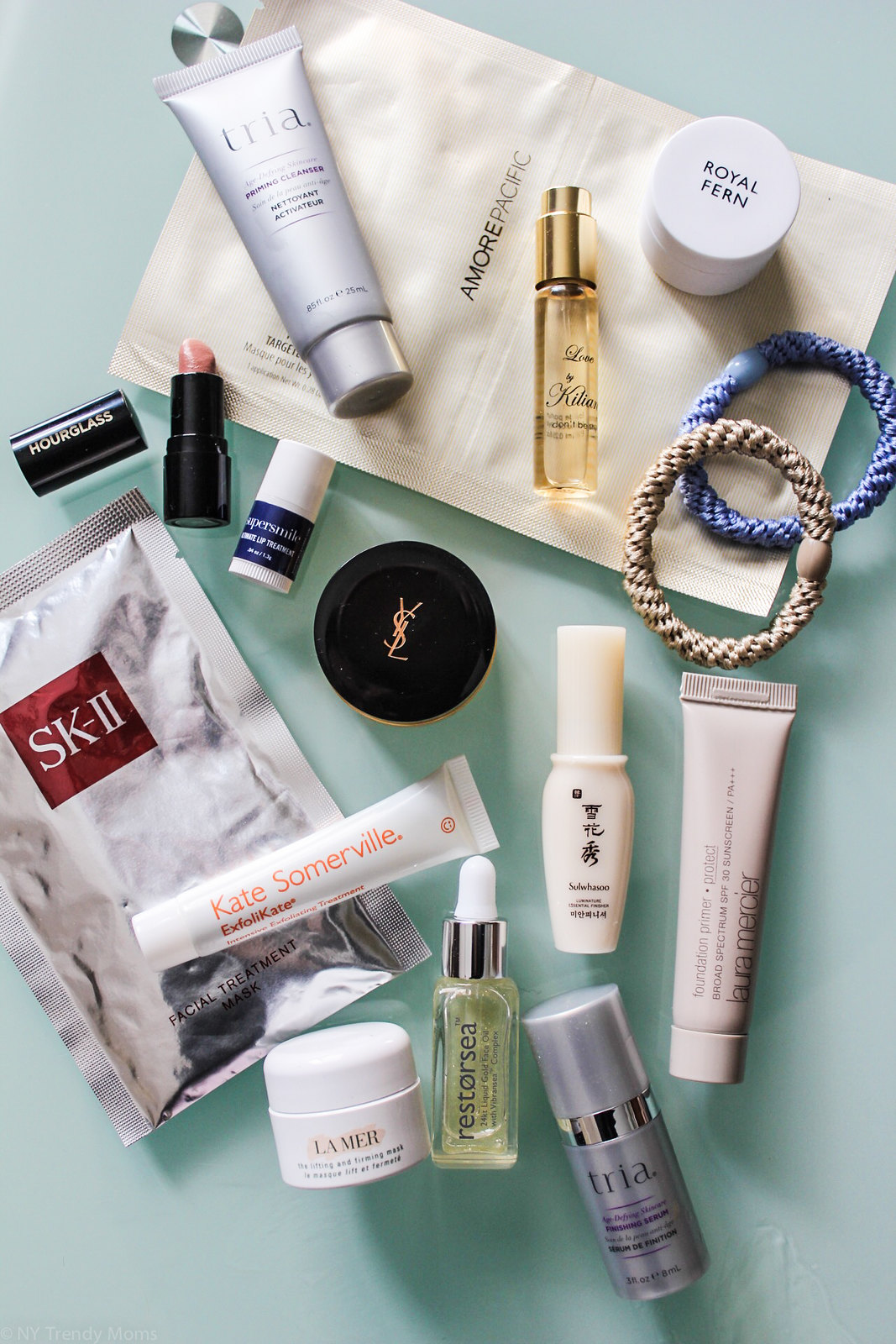This professionally styled product photograph showcases an array of sample-sized skincare and beauty products meticulously arranged on a light teal background. The composition evokes the feeling of a curated beauty box or subscription set. 

In the upper center, samples of shampoo and conditioner stand out, accompanied by another similarly packaged item in silver and red labeled "facial treatment." Renowned brands such as YSL, La Mer, Kate Somerville, and Hourglass are prominently featured. A small trial size perfume bottle adds a fragrance element to the collection. 

Additionally, two hair ties—one tan and one blue—are laid out, adding a practical touch. Notably, an Hourglass lipstick in a soft pink hue is displayed with its cap off and the lipstick twisted up, highlighting its shade. A tiny, sealed La Mer cream sample is also included, underscoring the luxury aspect.

Completing the set are various serums and oils, including one in a white container labeled "Royal Fern" and a visibly oily substance in another bottle, emphasizing a comprehensive skincare routine.